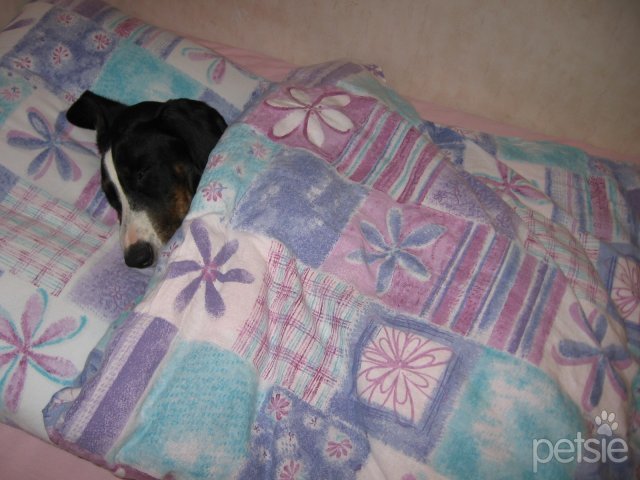This cozy indoor photo captures a sleeping dog tucked into a warm, colorful blanket. The dog's head, featuring a black nose, brown fur with a white stripe running down its forehead to its snout, and long ears—with one ear partially flipped up—rests at the top left corner of the image. The blanket, adorned with floral patterns and pastel colors of pink, lavender, white, and bluish-green, envelops the dog's body, making it appear snug and comfortable. In the bottom right corner, a watermark reads "Petsie," with a playful paw print dotting the 'I'. The room's wall, a whitish off-color, serves as a neutral backdrop to the heartwarming scene of the dog peacefully resting in a bed.